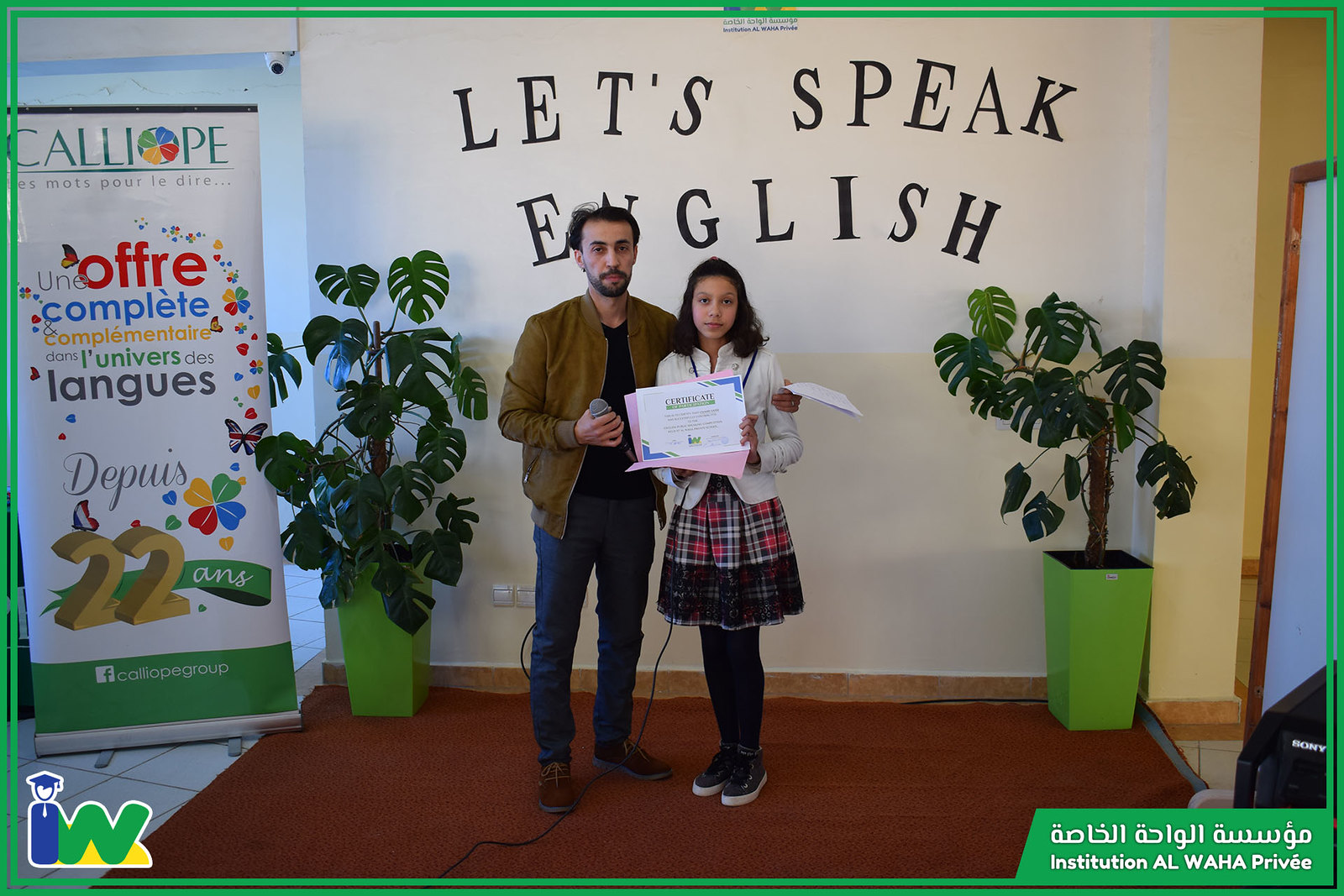This vibrant indoor photograph showcases a middle-aged man with dark hair, a black mustache, and a beard, dressed in a brown jacket, black shirt, and blue jeans. The man is holding a microphone plugged into the wall behind him. Beside him stands a young woman in her twenties, wearing a white jacket, a red, white, and black plaid skirt, black leggings, and black shoes. She holds a certificate, both smiling in front of a white wall featuring bold black letters that read "Let's Speak English." 

The background includes various details: a banner or poster mentioning "Calliope" and language offerings, hinting at an educational setting, possibly related to learning English. The scene is flanked by two large plants, adding a touch of greenery. A green border frames the photograph, and a watermark in the lower left corner bears the logo "IW," styled to resemble a graduate, along with text in English and Arabic, stating "Institution Al-Waha Privé." The image appears to celebrate an achievement or milestone in language education, captured in a moment of pride and shared accomplishment.